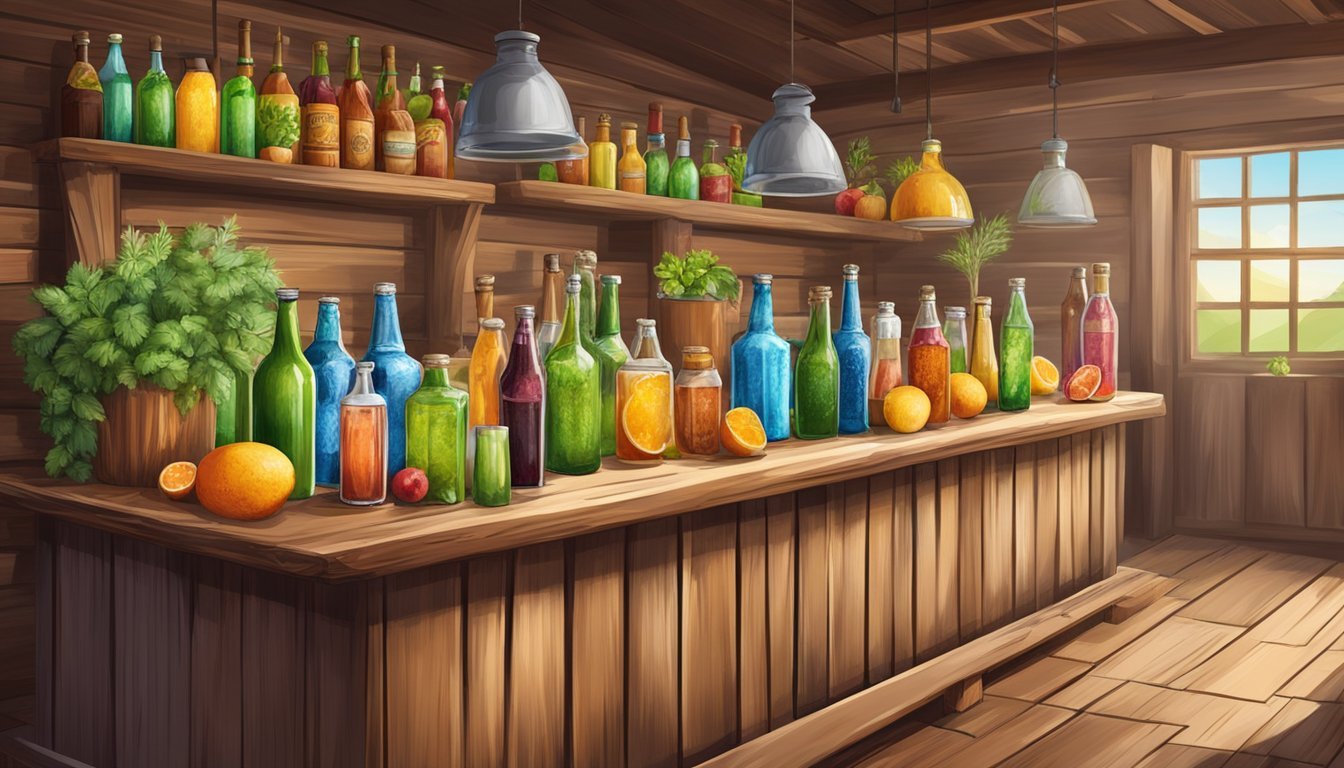The illustrated image depicts a detailed, cartoon-style wooden bar crafted from light-colored, unfinished wood that permeates the ceiling, walls, floor, and shelving. The bar, shaped in an L-formation, is adorned with an array of vividly colored glass bottles ranging in shapes and sizes, including green, blue, orange, purple, pink, and red bottles, some containing liquids of diverse hues. Interspersed with the bottles, there is an assortment of fresh citrus fruits such as grapefruits, oranges, and possibly a plum. On the left side of the bar sits a large potted plant, while additional smaller potted plants are positioned around the bar and suspended from the ceiling. The bar itself rests on a matching wooden plank floor, beneath four hanging glass lights—three clear and one orange—that dangle from the wooden ceiling. Behind the bar, a higher shelf echoes the display of multicolored bottles. The room features a single window, allowing natural light to enhance the rustic ambiance of the scene.